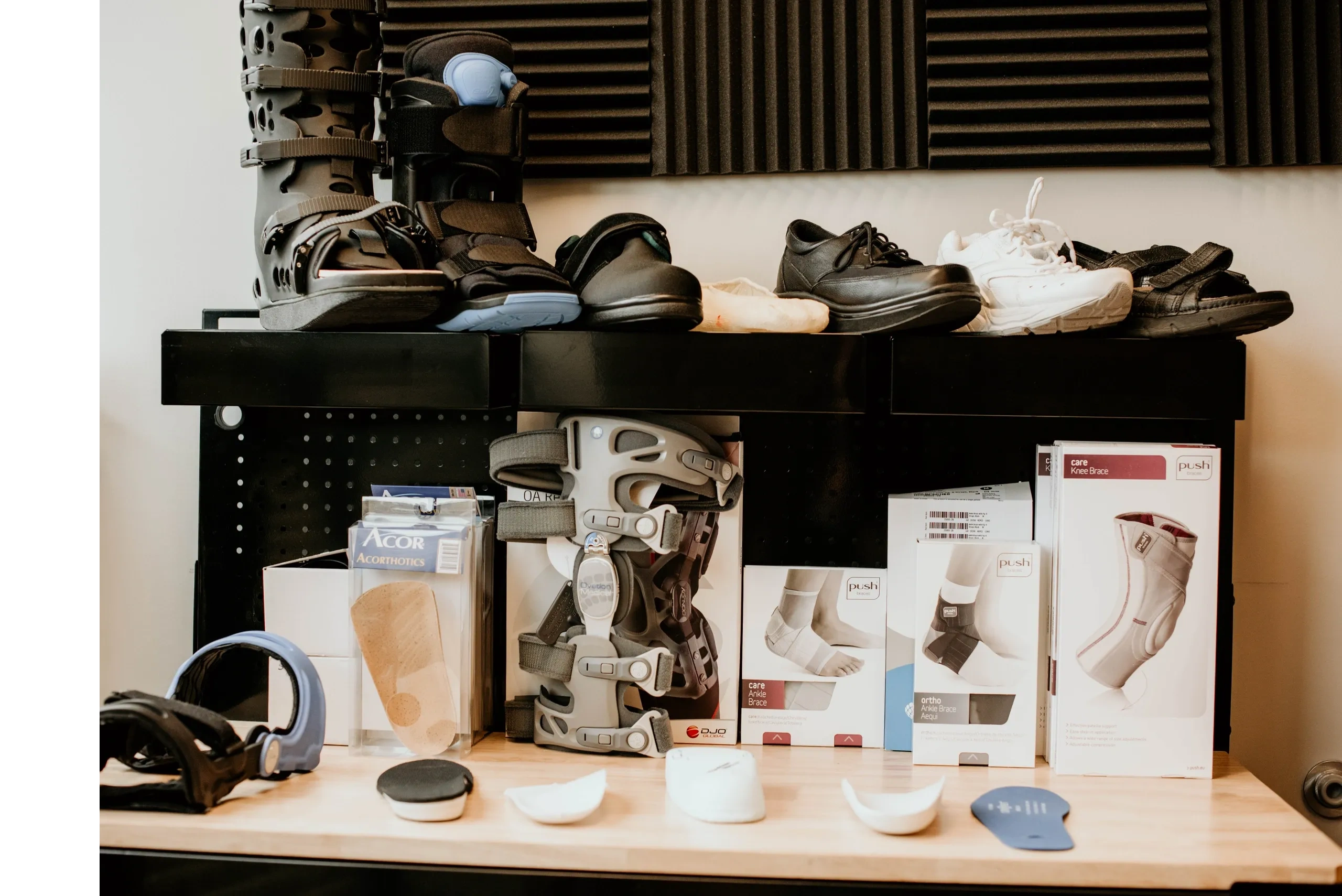This detailed photograph showcases an orthopedic display on a light-colored wooden table set against a white wall with four sound-dampening styrofoam panels. On the tabletop, various knee and ankle braces, as well as orthotic shoe inserts, are meticulously arranged. The table also supports a black shelf towards the rear, which holds six pairs of shoes and two orthopedic boots in different sizes. Specifically, the shoes include a black pair of sandals, a white pair of tennis shoes, a black pair of dress shoes, a pair of ballet shoes, an orthotic shoe, and two walking boots—the larger one on the left. The table is backed by a black pegboard and displays different knee and ankle braces. On the right side, there's a knee brace, followed by a black ankle brace, a white ankle brace, a more robust and buckled knee brace, and a package with a shoe insert. In front on the left side, there is a knee brace with a light blue powder coating. The array of orthotic shoe inserts in front ranges from thinner, curved styles on the left to thicker, more even designs in the middle, and a flatter blue orthotic on the right. Additionally, five white boxes containing ankle support braces enhance the organized display.